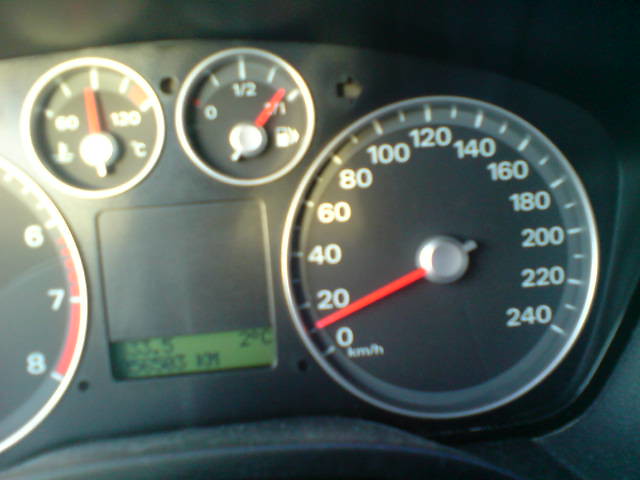The image depicts the dashboard of a vehicle, possibly a car or an airplane, although the exact type is unclear. The dashboard is predominantly black or gray. On the left side, there is a partially visible gauge, showing the numbers 6, 7, and 8, with a red mark next to these numbers. In the central part of the dashboard, there are two smaller and slightly blurry circular indicators. The first indicator has a red bar pointing nearly straight up, slightly to the left, while the second has its red bar positioned to the right side. The first indicator includes the numbers 0 and ½, suggesting it might be a fuel gauge, though part of it is obscured.

On the right side of the dashboard is a larger, clearer circular gauge labeled "km/h" for kilometers per hour. This speedometer displays numbers ranging from 0 to 240, with small marks indicating each increment. The red indicator bar on this gauge points at approximately 10 km/h, positioned between 0 and 20.

In the very center of the dashboard, there's a small, mostly obscured square area with a gray overlay. Behind this, a green screen displays some black numbers, although they are not clearly visible.